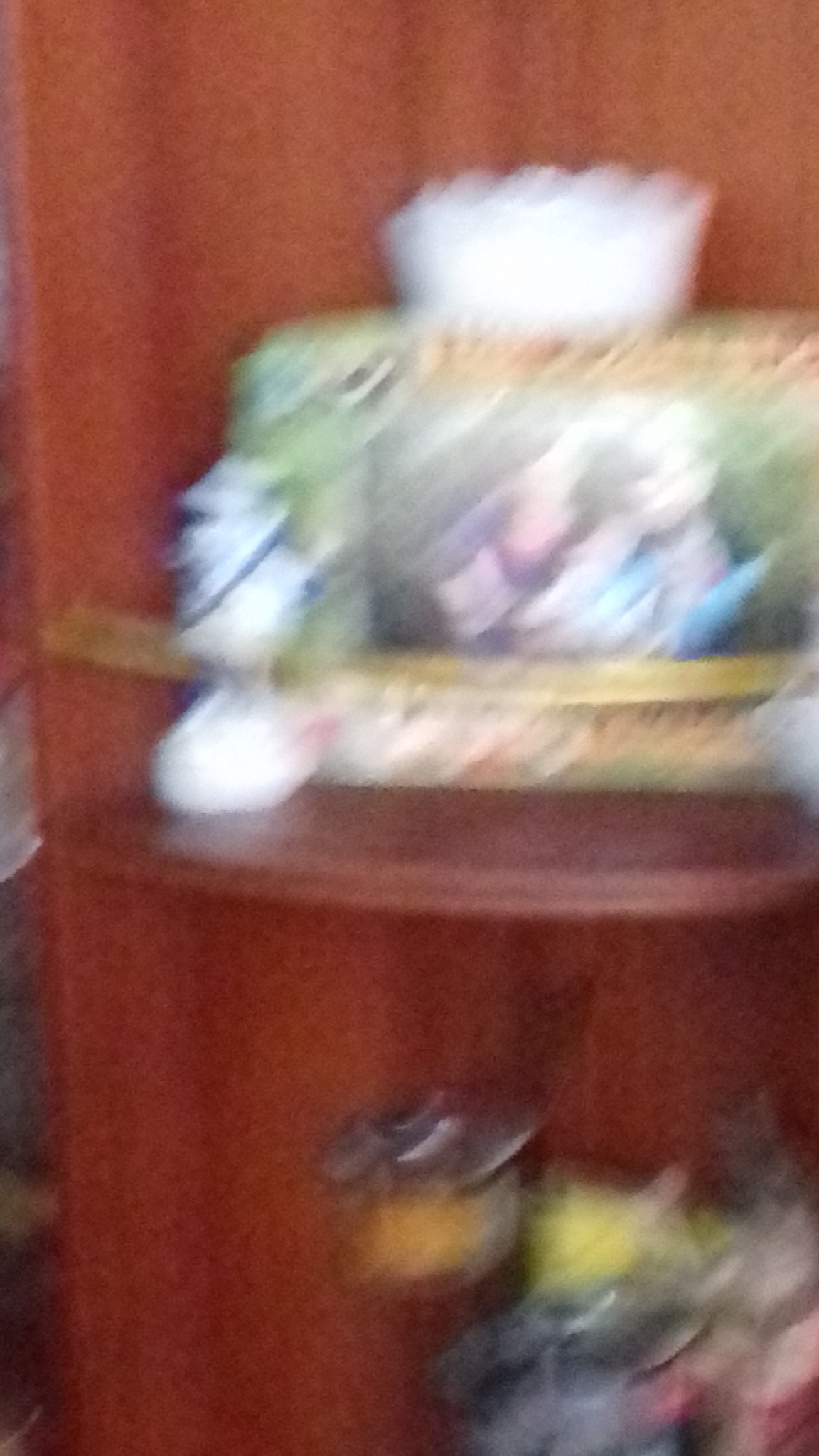The image portrays a blurry photograph capturing a single shelf adorned with various decorative items. The shelf appears to be constructed from a dark reddish-brown wood, imparting a warm and elegant ambiance. It has a modest, thin framework with a distinctive rounded design, resembling an open triangle or half of a square.

Positioned on the shelf is a vibrant but indistinct picture, its details obscured due to camera movement during the capture. The colorful nature of the picture suggests it is a vivid and eye-catching element of the display. In front of this blurred image, there are several small statues, adding a layer of ornate charm.

Below this main shelf, another similarly styled shelf hosts additional decorative pieces, including more colorful statues or figurines. The collective arrangement of these elements, despite the blur, evokes a sense of thoughtful and artistic decoration.